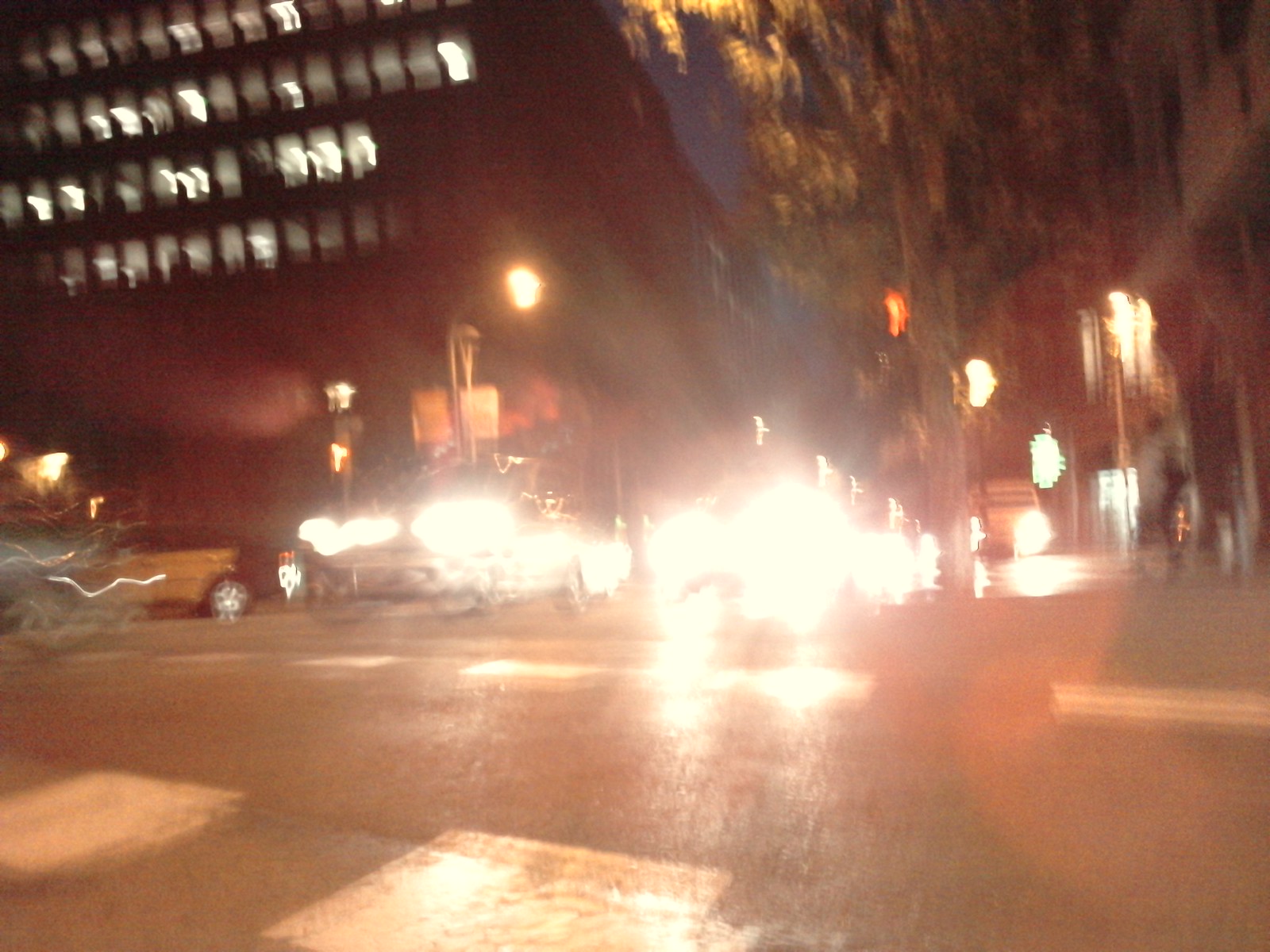A nighttime street scene, captured in landscape mode, is heavily out of focus and overexposed. In the top left corner, the windows of a multi-story skyscraper, at least four floors high, can be discerned. A stream of cars is moving towards the viewer from the left side of the frame, their headlights forming a bright, intense line. The foremost car to the left is distinctly visible as a yellow vehicle. A pedestrian walks towards the viewer on a dimly lit sidewalk that runs parallel to the street. The crosswalk is faintly visible at the bottom left corner of the photograph, accompanied by the glow of streetlights and traffic signals that add to the urban nightscape.